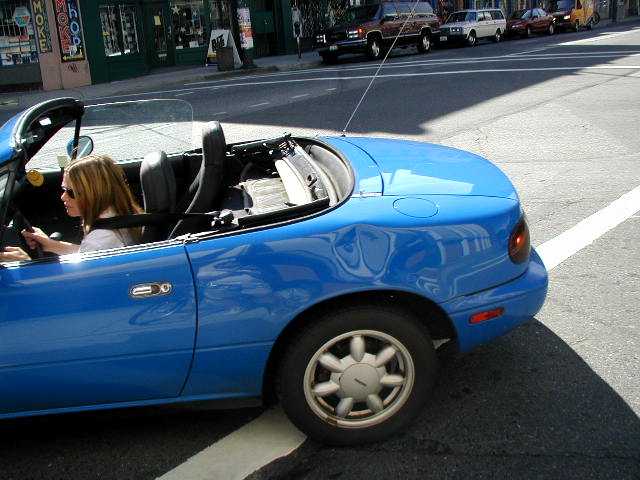In this image, a woman with long brown hair featuring blonde highlights is seen driving a bright sky blue convertible with a black interior. She is wearing black sunglasses and has both hands on the steering wheel. The top of the car is down, and she is secured with her seatbelt visible over her shoulder. The car appears to have a dent over the rear tire, although it could be a reflection. She is executing a sharp turn, crossing a solid white line, on an asphalt roadway in a city setting. The driver's side window is down, while the passenger side window is up. The background reveals a sunny day with her shadow cast on the foreground. A row of parked vehicles, including cars and SUVs of various colors, line the opposite side of the street adjacent to storefronts, advertising signage, parking meters, and a light pole. There is also a hint of a motorcycle reflected in the car's surface.